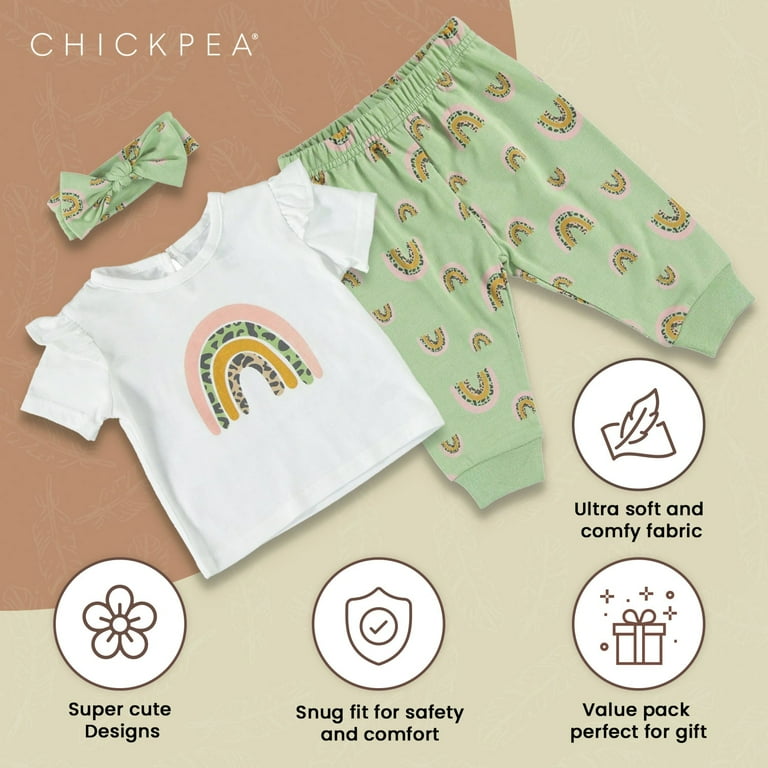This image is a detailed advertisement for a company called Chickpea, promoting an adorable children's clothing set. The background features a dark brown swoop in the upper left corner that transitions into a light greenish-gray area, providing a cozy and calming aesthetic. The prominent text "CHICKPEA" appears in all caps in the top left corner, accompanied by a trademark symbol.

Central to the image is a coordinated outfit likely intended for a little girl. The outfit consists of a short-sleeved white T-shirt adorned with ruffles at the shoulders and an eye-catching rainbow print in the center. The rainbow deviates from traditional colors, boasting a pink arc, a green leopard print arc, a light orange arc, and finally, a brown and black cheetah print arc. Complementing the T-shirt is a pair of light green pants with an elastic waistband and elastic leg cuffs. The pants are decorated with the same unique rainbow pattern, some of which are positioned upside down. Additionally, the set includes a matching light green hair bow featuring the same rainbow design.

Four informative circular icons are strategically placed around the outfit, highlighting its key features. The top right circle depicts a feather and paper, with the text "Ultra Soft and Comfy Fabric" underneath, emphasizing the comfort of the material. The bottom right circle shows a gift box with stars, proclaiming "Value Pack, Perfect for Gift," suggesting the set's suitability as a present. The bottom center circle has a shield with a check mark, indicating "Snug Fit for Safety and Comfort," assuring a secure and comfortable wear. Lastly, the bottom left circle with a flower icon declares "Super Cute Designs," underlining the outfit's charming aesthetic.

This Chickpea advertisement effectively showcases the detailed design and thoughtful features of their children's clothing set, making it an appealing choice for both parents and gift-givers.